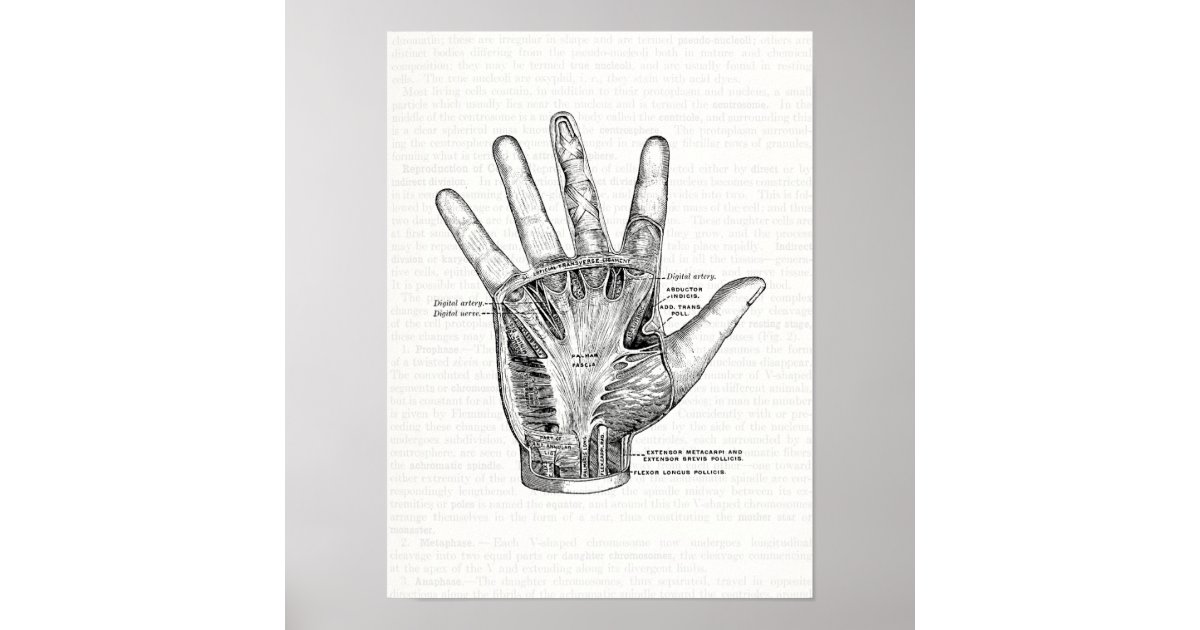This poster, predominantly black and white, features an intricate diagram of the anatomical structure of a right hand, palm side up with the thumb facing outward. The depiction varies in detail across the fingers: the pinky and ring fingers retain their skin, the middle finger is completely exposed showing muscles and tendons, while the index finger has a partially exposed section. The palm is entirely stripped of skin, revealing detailed tendons and muscles labeled with small call-out texts naming parts such as "digital artery" and "digital nerve." These labels are quite small and somewhat difficult to read. The diagram appears to be sourced from a medical or scientific textbook. Surrounding the hand, a pattern of faint and sheer text covers the white background of the poster, giving the impression of a textbook page. The overall poster rests on a gray background and has a slightly taller than wide rectangular shape.